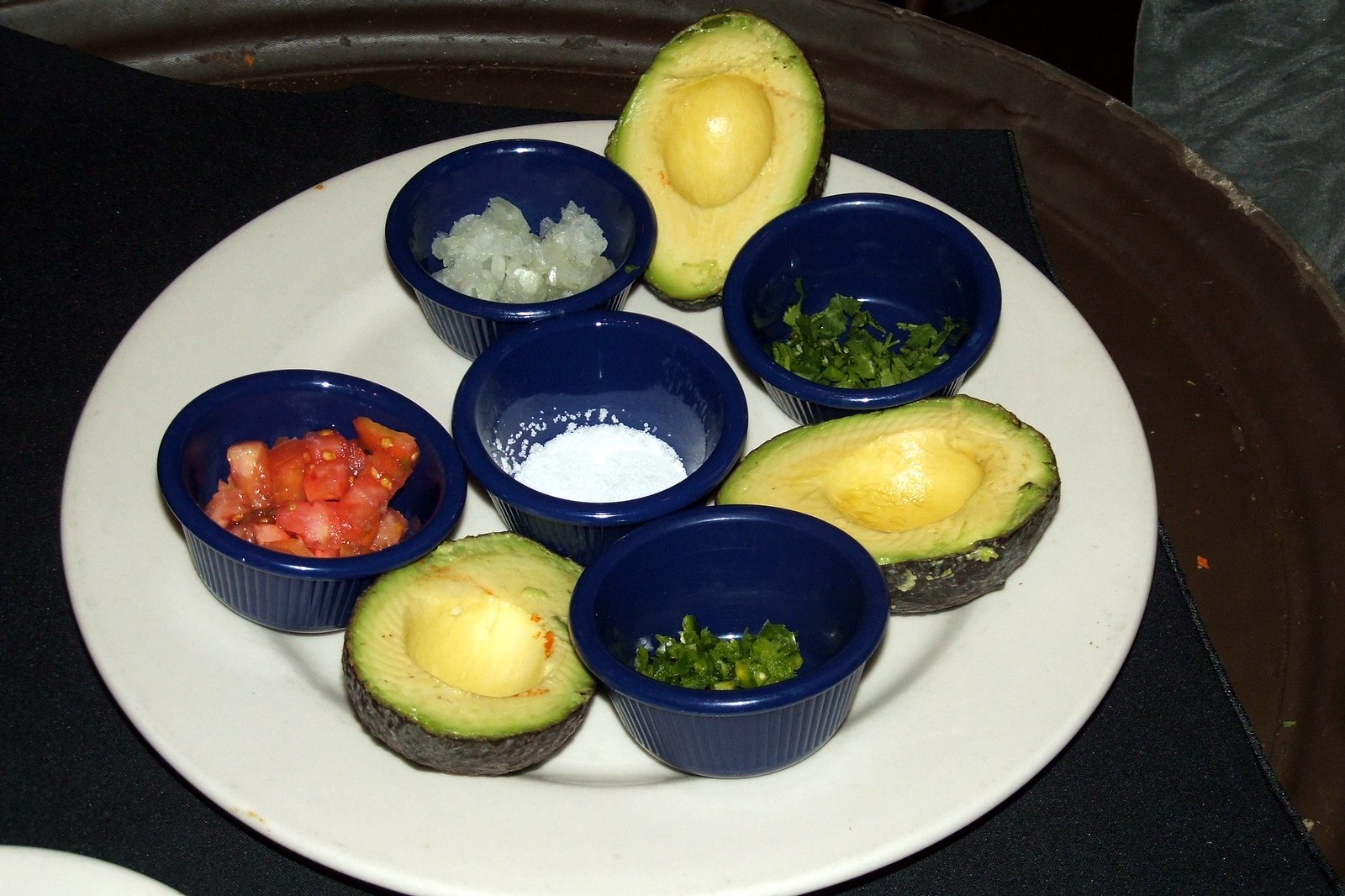The image depicts a wooden table with a black tablecloth on which rests a white dinner plate. Centered on the plate are three avocados, each cut open with their pits removed, but with the skin still intact. Surrounding the avocados, there are several smaller blue bowls, each containing various ingredients. One bowl holds diced tomatoes, another contains chopped onions, while a third has chives or cilantro. Additionally, one blue bowl in the center holds a white substance, possibly salt or cream. These items are likely arranged for preparing guacamole. The avocados, along with the vibrant colors and neatly arranged ingredients, suggest a fresh and inviting setup. There is also another plate partially visible in the left corner of the image.